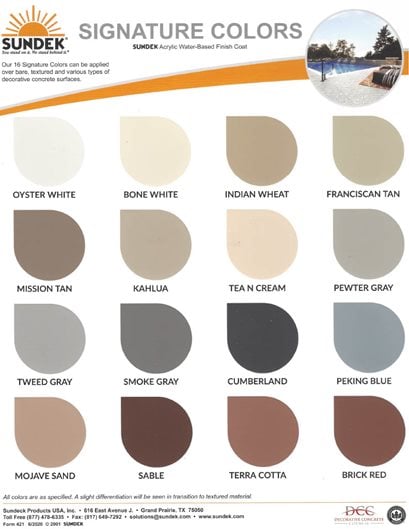The image displays a paint sample card typical of what you'd find in a hardware store, featuring a variety of color options for concrete surfaces. Set against a white background, the top of the card prominently includes the words "Signature Colors" in gray lettering. In the top left corner, there is a geometric sun logo in yellow, accompanied by the word "Sundeck" spelled out as S-U-N-D-E-K, with additional smaller, unreadable text beneath it.

On the left, a mustard yellow banner ending in a circular icon depicts a deck area surrounding a square swimming pool, suggesting an application context for the colors. Beneath this, the card showcases four rows of different shades of paints, primarily earth tones. There are sixteen paint samples in total, organized from left to right, top to bottom:

1. Oyster White – a bare white shade.
2. Bone White – a cream-colored sample.
3. Indian Wheat – a brown tone.
4. Franciscan Tan – a grayish tan.
5. Mission Tan – a brownish tan.
6. Kahlua – a grayish tan.
7. Tea and Cream – a pinkish tan.
8. Pewter Gray – a basic gray.
9. Tweed Gray – a bluish gray.
10. Smoke Gray – a dark gray.
11. Cumberland – almost black.
12. Peking Blue – a light blue.
13. Mojave Sand – a pinkish brown tan.
14. Sable – a dark brown.
15. Terracotta – a medium pink brown.
16. Brick Red – a reddish-brown leaning towards brown.

Below the color samples, there is small black text, but it is too fine to decipher. The card appears to be from a company offering these signature colors for concrete surfaces, promoting their acrylic water-based finish coat suitable for various decorative applications.